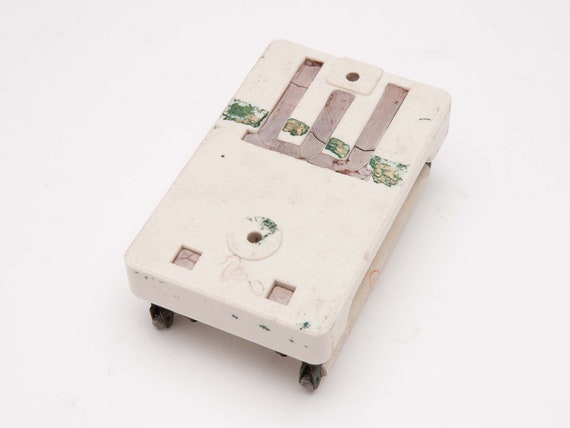The image captures a professionally taken photograph of a white rectangular device positioned on a white surface, viewed from a slight angle above and in front. The device, resting on black rails or legs, showcases a minimalist design featuring multiple geometric elements and colors.

There are prominent light purple and green lines decorating the device, as well as three vertical gray columns, which span from the top to the middle and are connected by a horizontal gray line. Two small gray squares are positioned near the bottom edges, equidistant from each other, just below a circular feature at the lower part of the rectangle. At the very top center of the device, a small circular hole suggests a lens, akin to those found on cameras or smartphones. The overall color palette includes black, white, brown, green, light purple, beige, and tan, which adds a visually engaging contrast amidst the clean, white background.